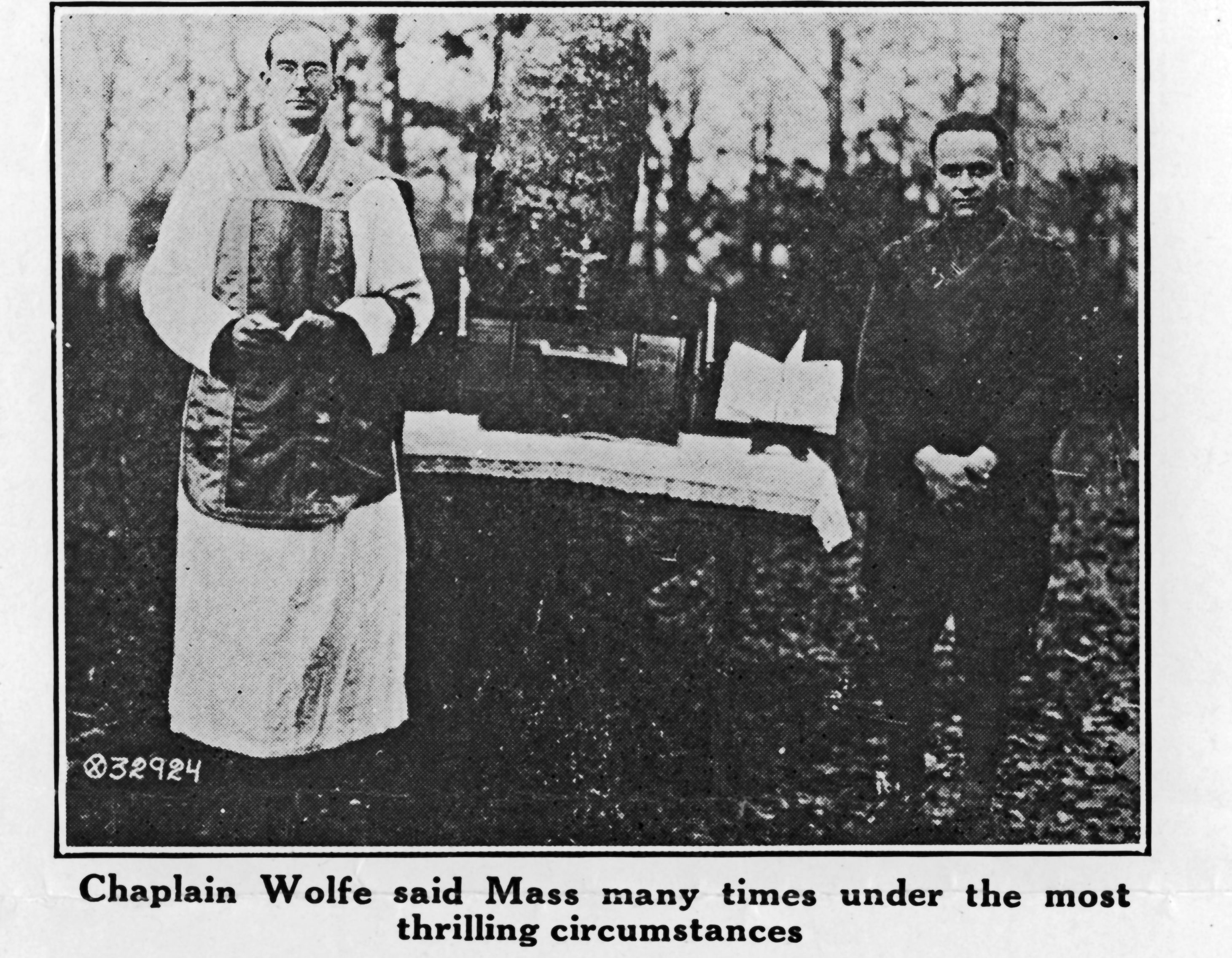In this very old black and white photograph, two men stand in a forest surrounded by trees with bare branches and a forest floor covered in leaves. The man on the left, referred to as Chaplain Wolf in the caption, appears to be religious, dressed in white clerical robes with a black apron-like garment over them. He has short hair, glasses, and no facial hair. To his right, there is a table draped with a white cloth featuring crosses and other religious artifacts, resembling an altar. A book holder with an open book and a cross flanked by two candles adorn the table, which is positioned in front of a tree. The second man, standing to the right of the table, is dressed in all black, with short hair and no facial hair. He stands with his hands clasped in front of him, both men gazing at the camera. The photograph is bordered by a solid white frame with a thin black outline, and in the lower left corner, there is an X in a circle followed by the numbers 3, 2, 9, 2, 4. Beneath the image, the black text reads, "Chaplain Wolf said mass many times under the most thrilling circumstances," indicating the chaplain's dedication to his duties even in such surroundings.